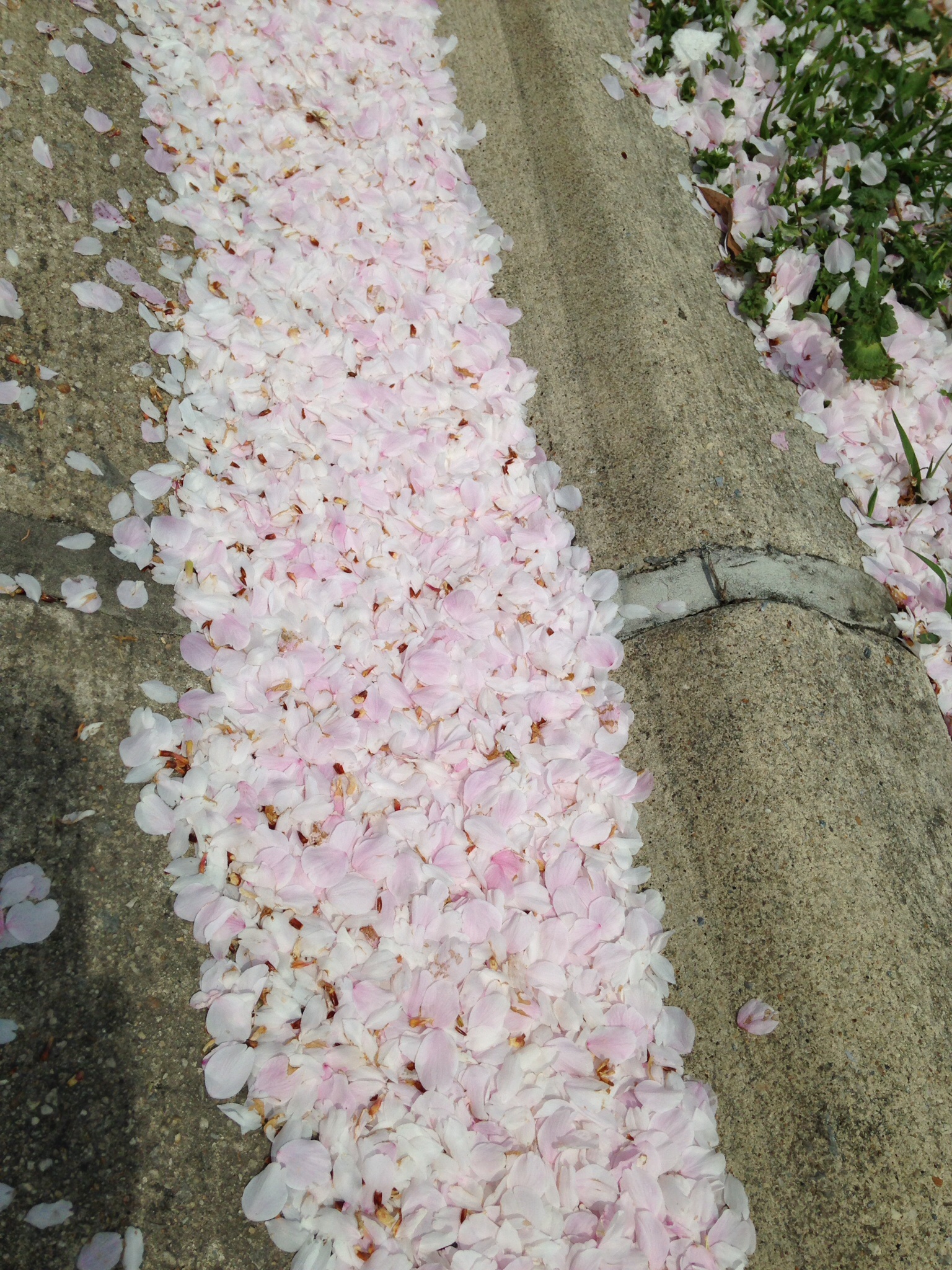This outdoor daytime color photograph captures a sunny scene where the curb meets the street, showcasing the aftermath of cherry blossoms shedding their petals. In the upper right corner of the image, a myriad of white to pink cherry blossoms, accompanied by green grass, cascade down to the middle right of the photograph. These blossoms blanket the ground alongside the curve, where the curb, made of cement, arcs gently. The left side of the curb is adorned with a dense accumulation of the petals, creating a visual flow from the top down to the bottom right of the image. Prominently in the center, a gray segment lies horizontally across the cement curb, delineating a joint where two large concrete pieces meet. Adding to the intricate details, a shaded area in the bottom left suggests the presence of the photographer, subtly casting a shadow over the scene. Overall, this close-up vividly portrays a charming springtime phenomenon, with cherry blossoms blanketing a concrete gutter.